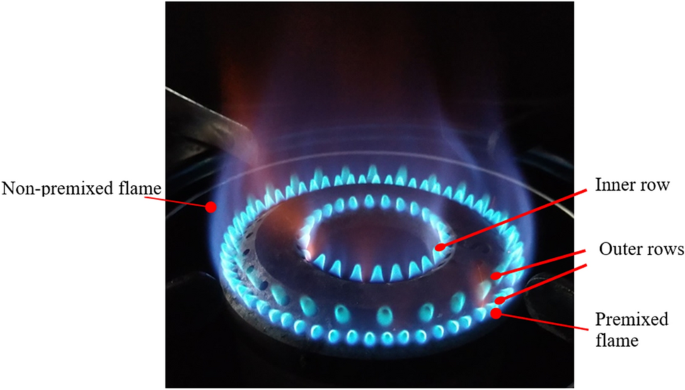The image depicts a detailed diagram of a blue flame burner, likely a stovetop or heating element, set against a black background. The burner consists of several concentric circles, each with aligned openings from which the blue flames emanate. These flames cast a bluish-purple glow upwards, indicating the high heat they produce. The diagram features red lines ending in red dots, which serve as arrows to label various components in black text, such as "non-premixed flame," "inner row," "outer row," and "premixed flame." The background includes faint, black metal pieces that are part of the burner’s structure, enhancing the dark contrast with the vibrant flames.